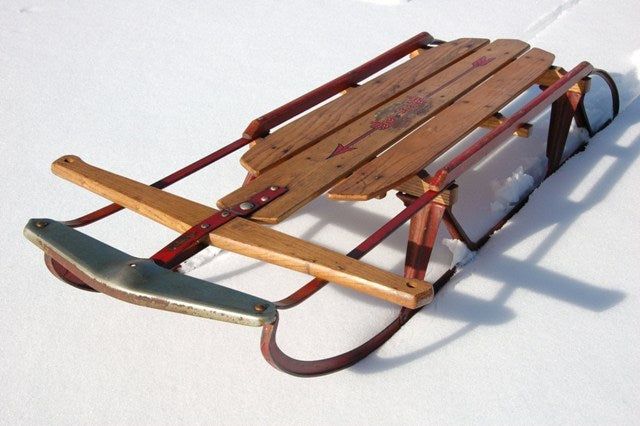The image depicts an old-school wooden toboggan sled captured from an angled perspective, showcasing both the front and top views. The rectangular photograph, whose top and bottom sides are twice as long as the left and right sides, features the sled cutting through a pristine blanket of flat, untouched snow, except where the sled's railings have left indentations in the top right corner. The toboggan itself is crafted from wood, with three distinct wooden planks forming its top surface, where one plank in the center is longer than the others. The sled's sides are flanked by heavy-duty metal railings painted in a worn red, revealing the blackened metal beneath. At the front of the sled, a large, triangular metal piece, likely serving as a protective bumper, is prominently visible. The toboggan features metallic elements, including large silver nails and screws, solidifying its robust construction. This detail-laden image emphasizes the nostalgic charm and enduring build of the vintage sled as it makes its way through the snowy landscape.